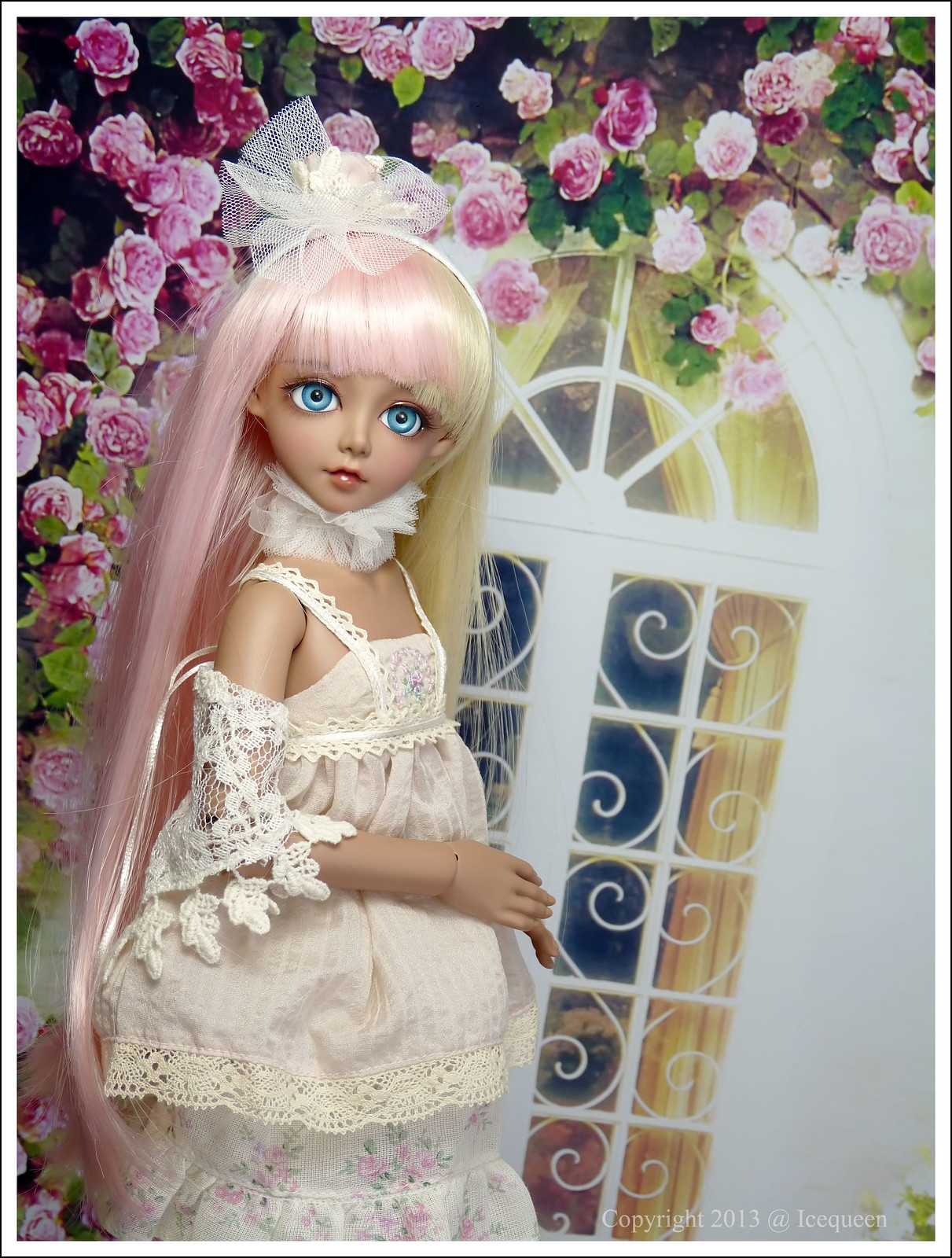This photograph captures a detailed portrait of a child’s toy doll with an intriguing blend of vivid colors and intricate details. The doll has an enchanting appearance, with long, flowing hair that is pink on one side and blonde on the other, cascading down past its hips. The doll’s large blue eyes are gazing directly at the viewer, with its head slightly turned towards the camera while its body faces to the right. The doll is dressed in a delicate white dress with thin straps, adorned with frills along its edges and hems, and it features see-through embroidered cloth around its arms. A frilly, white collar graces its neck, complementing the dress.

The background of the photo features a sophisticated setup that adds elegance to the doll’s appearance. The doll stands in front of a multi-paned, rectangular window with a distinctive arched top, which resembles a church window. This window is adorned with lush pink roses and green foliage forming an upside-down U-shape from the bottom to the top right corner, against a backdrop of gold curtains at the top panes. There's a marking in the bottom right corner of the image with the text “Copyright 2013 Ice Queen”. The overall composition of the photograph creates a whimsical and somewhat ethereal atmosphere, placing emphasis on the doll's striking features and elegant attire.